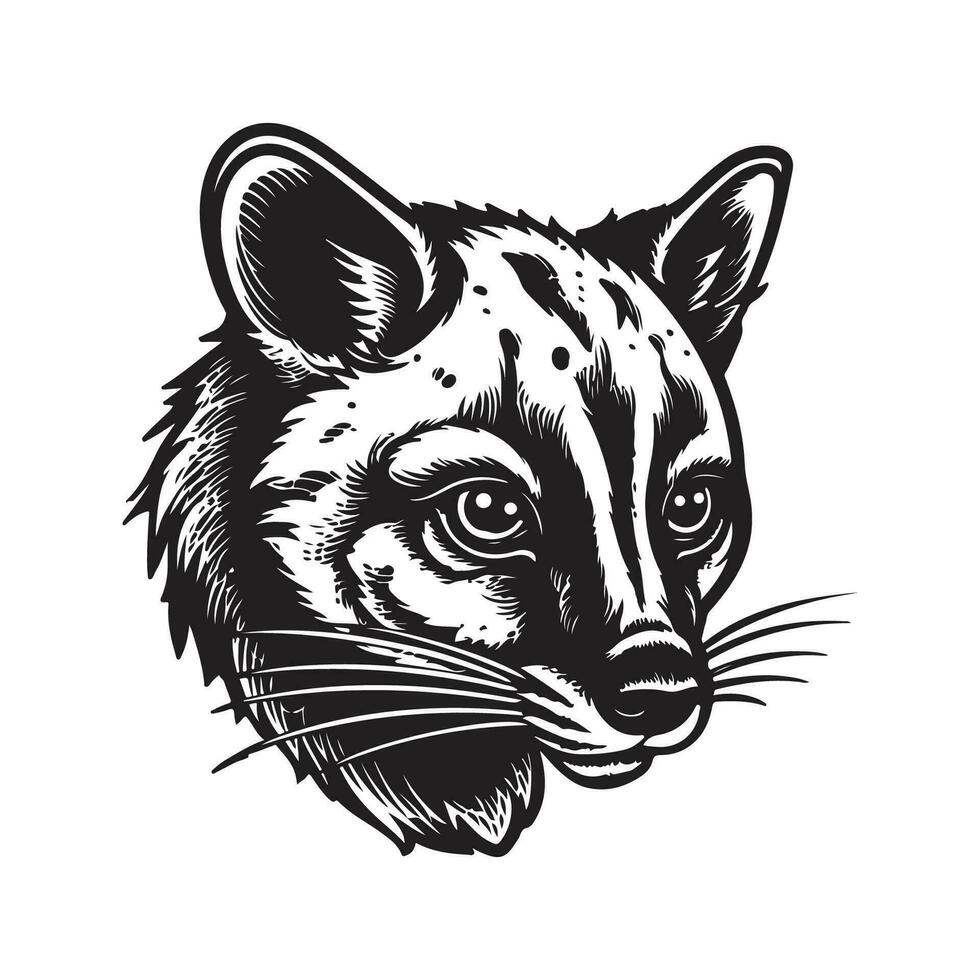This black and white illustration appears to be a stylized logo or emblem featuring an animal that resembles a fox, possibly a cat, or even a small dog or raccoon. The drawing highlights the animal's head, characterized by long whiskers on both sides, small steady ears, and large black eyes with two white dots in them. The face stands out as predominantly white against the dark surrounding features, with the black used to define the animal’s distinct characteristics. The simplified yet detailed artwork suggests it was created with a marker, pencil, or paint, and captures the essence of the animal with a focus on its expressive facial features. The animal glances to the right, adding a sense of intrigue and curiosity to the overall composition.